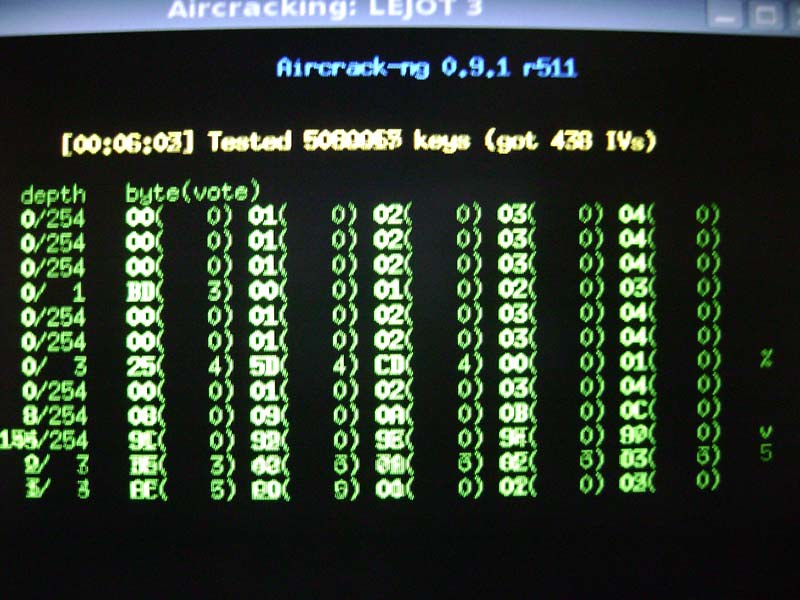The image depicts a black computer screen resembling a retro 1980s interface, showcasing the Aircrack-NG software version 0.9.1 R511 at the top in blue text. Below that, a highlighted line in yellow details "000603 tested 5080065 keys got 438IVs." Beneath this, rows of green text are organized into columns labeled "DEP," "byte," and "vote," displaying extensive sequences of numbers. Each number is part of a structured format, often repeated and followed by zeros, creating a dense matrix of digits. On the far left of the screen, beneath a percentage symbol, they indicate a value "V5." The overall layout and the pixelated font add to the retro feel, emphasizing the classic computer language aesthetics. The screen is an in-depth representation of Aircrack-NG's data-cracking process, showcasing comprehensive cybersecurity analytics.